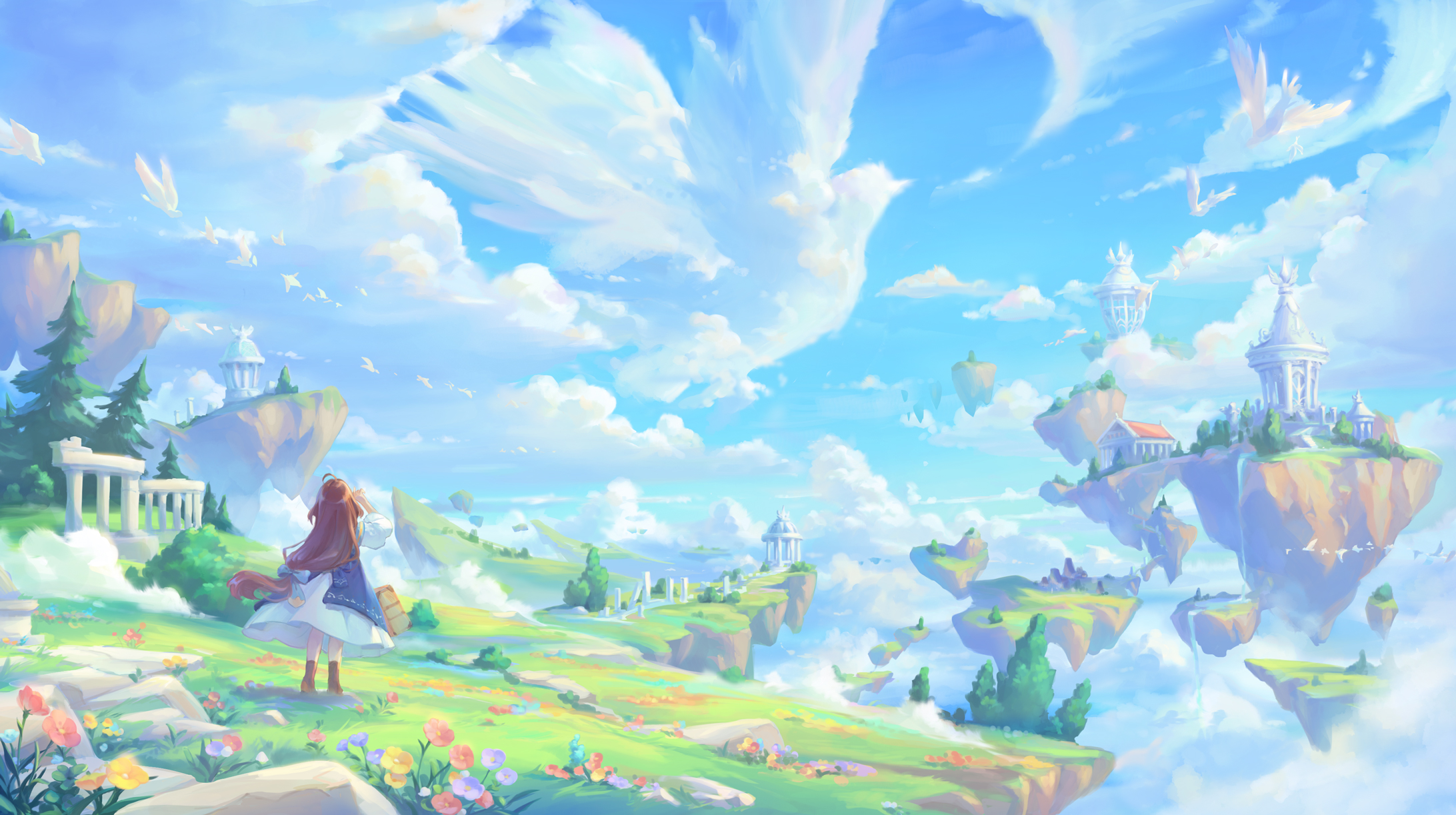The image is a detailed painting of a fantastical, anime-style world with floating islands suspended in a bright, colorful sky. These Earth-like islands, adorned with lush green grass and vibrant flowers, drift amidst puffy white clouds that resemble large birds such as swans or doves. Central to the composition is a young girl with long, dark brown or red hair cascading to the middle of her back. She stands on an island, gazing upward towards the sky. 

The girl is dressed in a blue blouse and a white, puffed-out skirt, complemented by brown ankle-high boots. She carries a small bag, adding to her whimsical appearance. The landscape around her is enchanting, with lush lawns, multicolored flowers, and structures like white pillars that may form part of a fence.

On one of the distant floating islands, there is an enchanted castle shrouded in clouds, while another island features a colosseum-like building with a distinctive red roof. In the distance, a lighthouse or lantern can be seen perched atop a rocky hill. The overall scene is bathed in bright and vibrant hues of greens, blues, reds, and yellows, accentuating the dreamlike quality of this otherworldly realm.